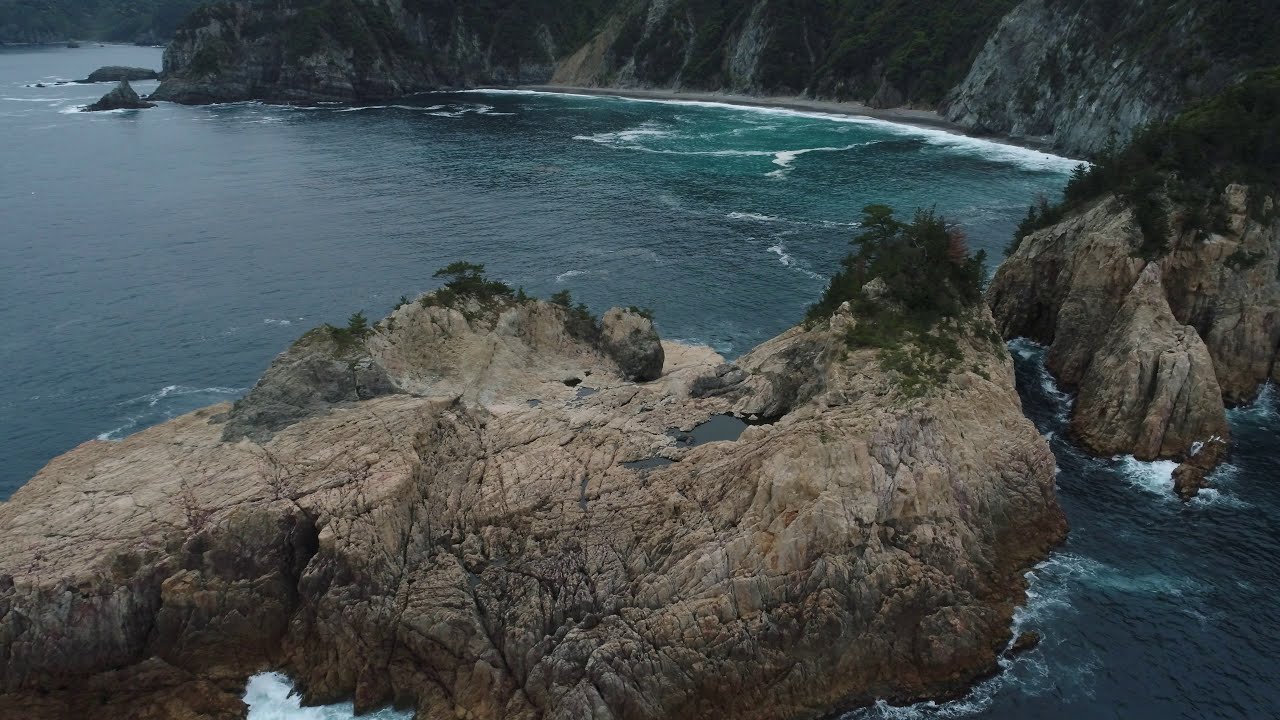This digital photograph captures a breathtaking aerial view of a coastal cove, framed by a horseshoe-shaped land formation that extends into the ocean. The scene is characterized by crystal dark aqua blue waters that transition into lighter shades in certain areas, reflecting the sun's rays. Waves crash onto a brown sand beach and against various rocky outcrops that surround the cove with hues of gray and brown. The rugged landscape is dotted with patches of green vegetation, including trees and bushes, particularly on the small rocky islands that punctuate the coastline. Despite the vibrant natural elements, there is no sign of human or animal life. In the background, the imposing mountains enshrouded in more greenery add to the dramatic scenery, completing this picturesque and untouched coastal vista.